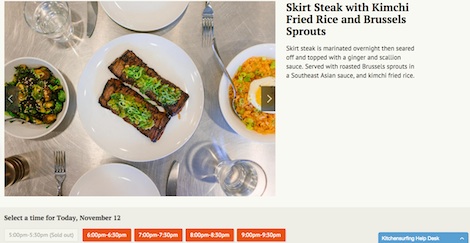This image is a screenshot from a website showcasing a specific dish: skirt steak with kimchi fried rice and Brussels sprouts. On the left side of the image, there is a photo of the meal, which is arranged on a stainless steel table along with some glassware and silverware. The right side features text detailing the dish. The name of the meal is prominently displayed with a description underneath explaining that the skirt steak is marinated overnight, seared, and topped with a ginger and scallion sauce. It is served alongside roasted Brussels sprouts with a Southeast Asian sauce and kimchi fried rice. Below the meal description, a section allows users to select a reservation time for today, November 12th. Various time slots are listed: 5 p.m. to 5:30 p.m. (which is sold out), 6 p.m. to 6:30 p.m., 7 p.m. to 7:30 p.m., 8 p.m. to 8:30 p.m., and 9 p.m. to 9:30 p.m.